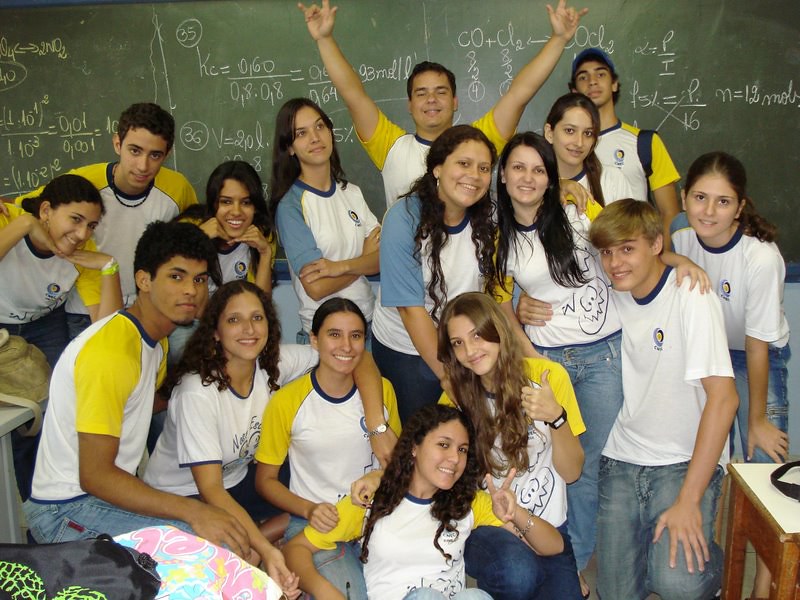This image captures a vibrant group of 16 teenagers, likely high school students, posing happily in front of a green chalkboard covered with various equations and chemical notations. The group consists of both boys and girls, with a mix of some standing, some sitting, and others kneeling. Most of them are wearing matching white T-shirts with either yellow or blue sleeves, adding a sense of unity to the scene. Visible in the bottom left corner are a black bag and a multicolored bag, while the bottom right corner shows a slightly out-of-frame wooden stand. The students take up almost the entire horizontal, rectangular photo, with some of them giving thumbs-up signs and one student in the back center triumphantly raising both arms in the air. Their wide smiles and cheerful expressions suggest a joyful moment, possibly within a classroom setting.